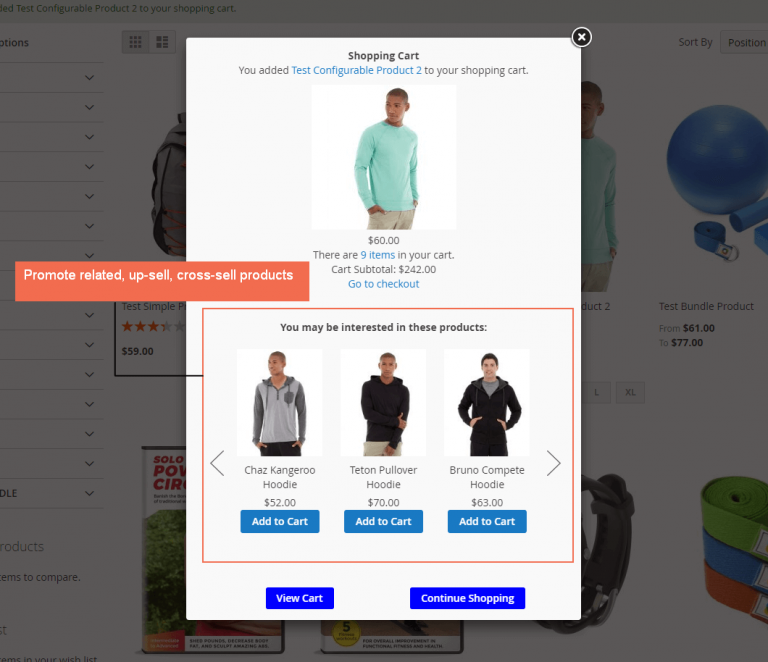This screenshot captures an online shopping experience with a detailed view of the shopping cart and related product suggestions. Here, we see a close-up of a section featuring an African-American model dressed in a light green shirt paired with white pants. The highlighted product, a light green shirt, is priced at $60. The user has added this item, described as a "test configurable product," to their cart, which already contains nine items bringing the subtotal to $242. 

At the top of the screen, there is a notification confirming the addition to the shopping cart, along with an option to proceed to checkout. Below this section, a "You may be interested in these products" banner showcases three hoodie options: the Chaz Kangaroo Hoodie, the Test Pullover Hoodie, and the Bruno Complete Hoodie. The models showcasing these products appear to be diverse, with two possibly being African-American and one either Hispanic or White. The hoodies are priced at $52, $70, and $63 respectively. 

Lastly, there are interactive buttons prompting the user to "View Cart" and "Continue Shopping." Partially visible in the background, there are other product listings, although they are obscured and not clearly identifiable. This snapshot effectively focuses on promoting related products and encouraging further purchases.